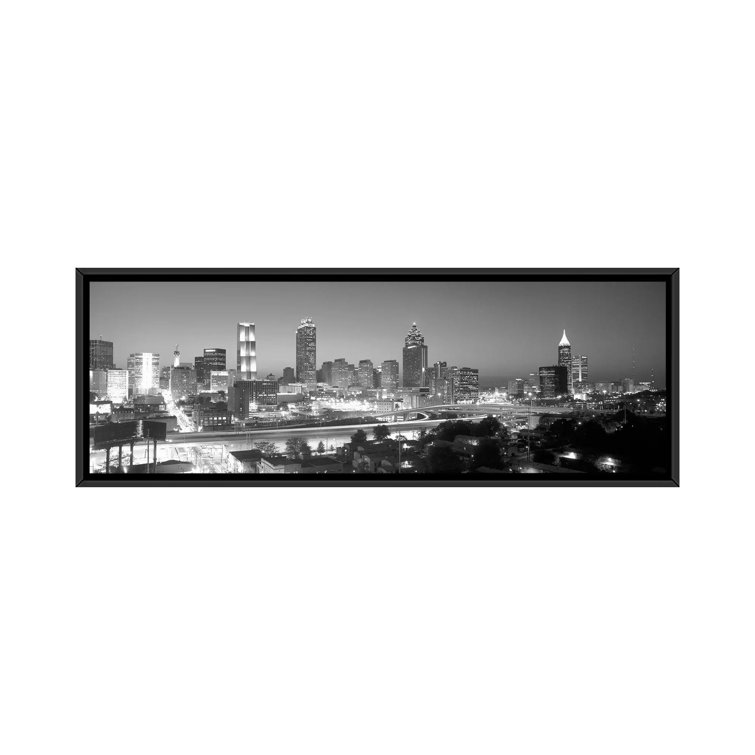This black and white, horizontal photograph, showcased within a thin black frame against a white background, captures a nighttime cityscape. Dominated by a skyline of towering skyscrapers, the city is half illuminated by the glowing white lights of numerous buildings, contrasting against the dark gray sky. Spanning the middle of the image, an extensive highway network is visible, featuring cloverleaf turns, bridges, and stretches of traffic that brighten the roadways. In the bottom left corner, the back sides of several billboards are discernible, while the lower right portion features trees and hedges, juxtaposing elements of nature against the urban vista.